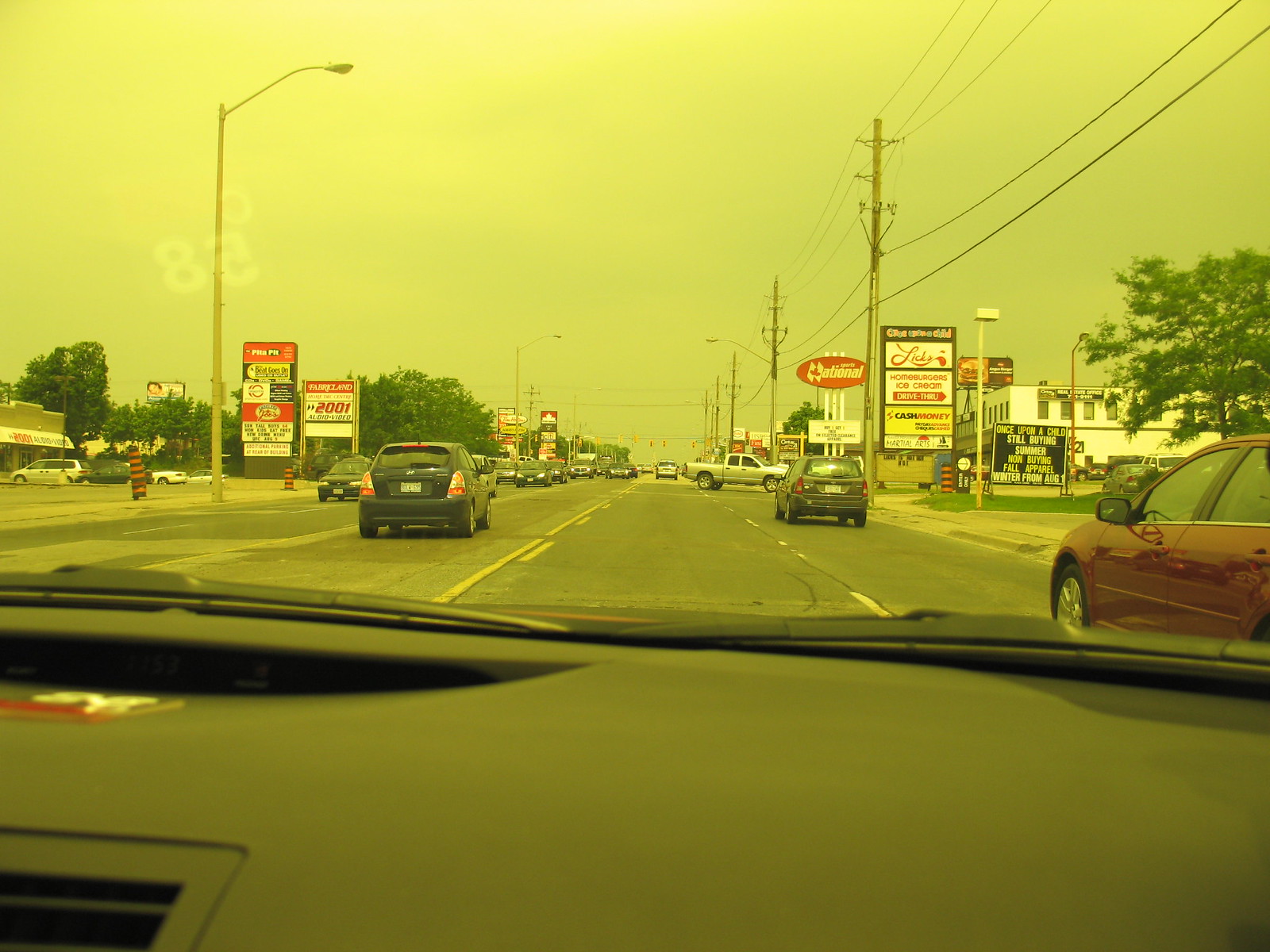An interior view from a car or dashcam captures the scene over a dark gray dashboard, presenting a multi-lane road. On the right-hand side, two lanes of traffic head in one direction, while an adjacent turn lane in the center is distinctly marked by yellow lines. To the left, two lanes cater to oncoming vehicles. The road is populated with various cars including blue, gray, silver, and red ones. The sky presents an overcast ambiance, imparting a subtle yellow tint to the overall image, likely due to the camera's settings. Billboards in white, red, and yellow hues line the roadside along with several storefronts visible on both sides.